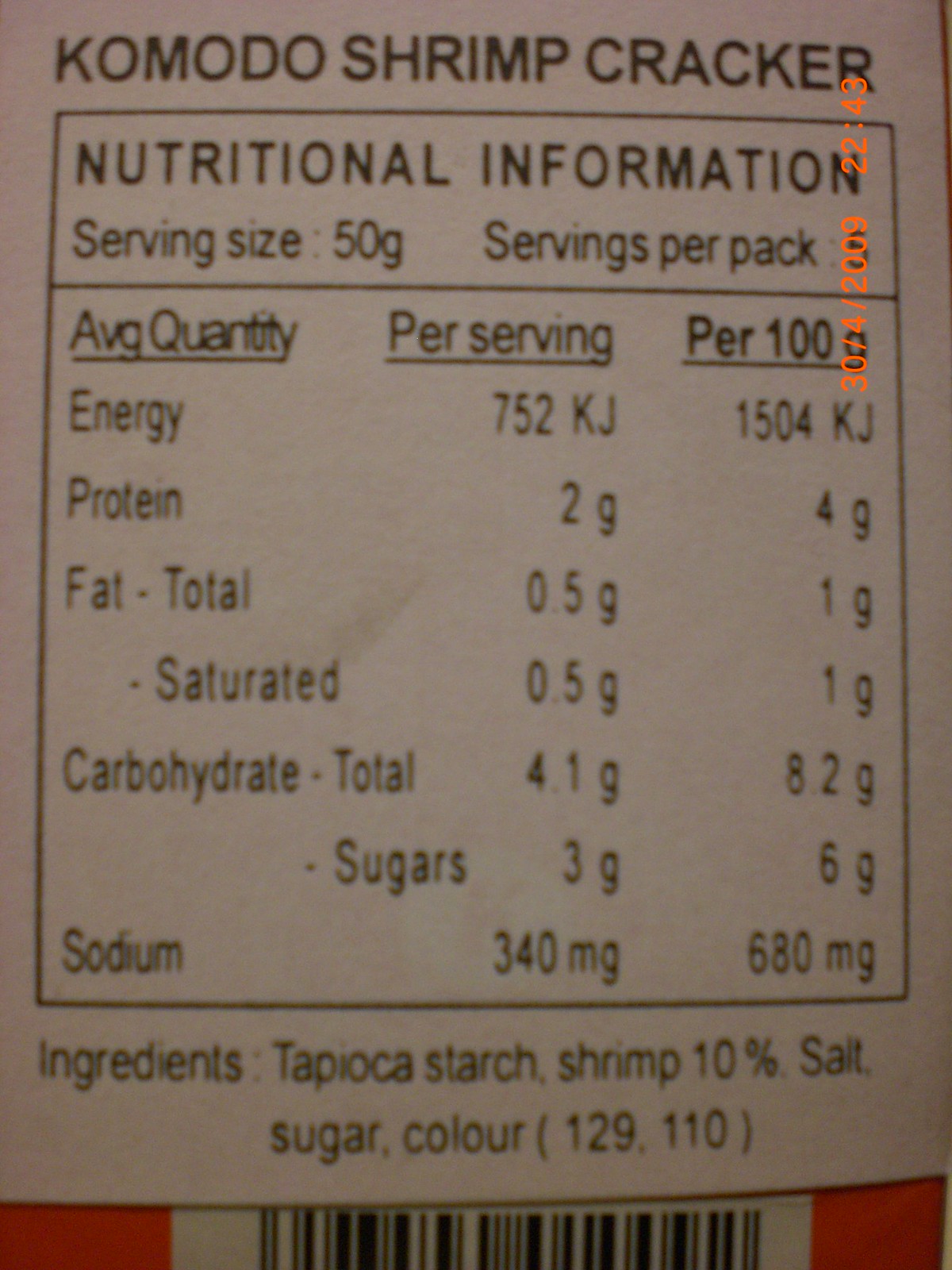The image is a photograph of a nutritional information label for Komodo Shrimp Crackers, set against a brown paper backing with black text. The label includes a detailed breakdown of nutrients with both per serving and per 100 grams metrics. Serving size is indicated as 50 grams, with multiple servings per pack, though the exact number of servings is obscured by a date and time stamp (30/4/2009 at 22:43) on the image. Key nutritional values per 50-gram serving include: 172 kilojoules of energy, 2 grams of protein, 0.5 grams of total fat (all saturated), 4.1 grams of carbohydrates (3 grams of which are sugars), and 340 milligrams of sodium. Ingredients list is tapioca starch, 10% shrimp, salt, sugar, and color additives. The bottom of the label features a barcode on a red background.